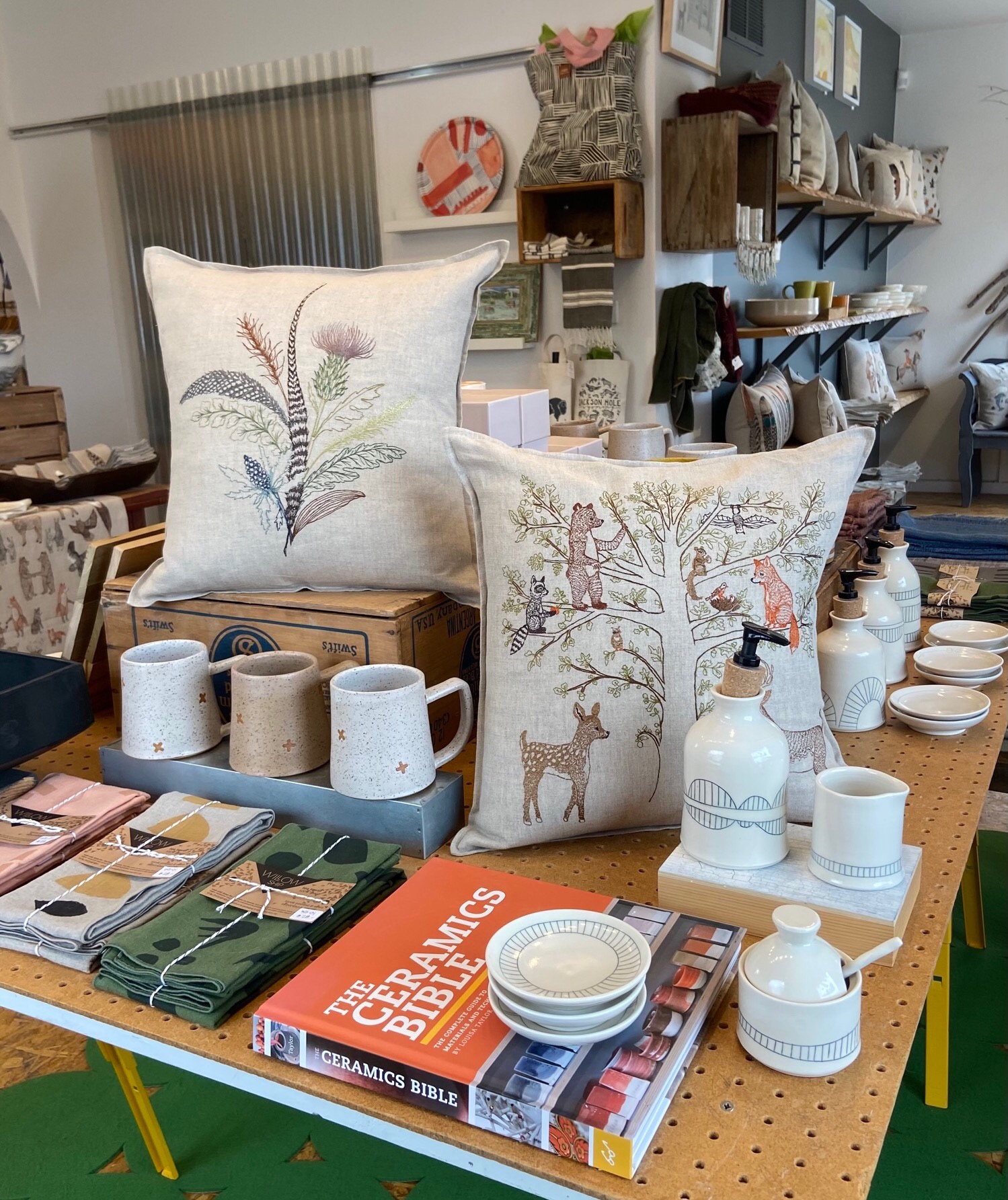This detailed photograph depicts the interior of what appears to be either a domestic setting or a craft shop, filled with artisan-made items. Central to the image is a unique table featuring a pegboard surface, typically seen on walls but interestingly repurposed here as a tabletop. The table is adorned with various handcrafted goods, including two throw pillows, multiple coffee mugs, jars, saucers, and napkins tied with twine. There are also soap dispenser-like bottles, coasters, and a notable orange book with white text titled "The Ceramics Bible." The ceramics, which are entirely white with lined geometric patterns, suggest a consistent craft theme. The background is bustling with additional shelves displaying more handcrafted items such as pillows, cutlery, cups, and other artisanal crafts, giving the scene a vibrant, busy atmosphere that could be indicative of a shop or an elaborate craft fair display.